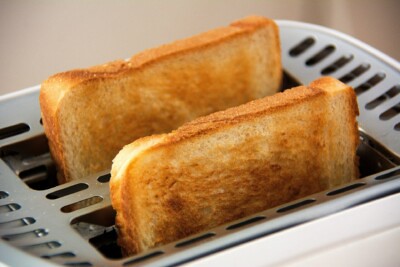This is an indoor, close-up color photograph of a toaster with two perfectly toasted slices of plain white bread, partially emerging from the slots. The toaster features a sleek design with white sides and a chrome top, characterized by oval milled holes. The bread exhibits a golden brown hue, darker toward the center with crisp, lighter edges, and appears to be commercially purchased white bread, evenly toasted without any special features. The background is out of focus with a tannish-brownish and white blur, suggesting an indoor setting. Notably, the toaster looks pristine with no visible crumbs, indicating it might be a new appliance or part of a staged product image.